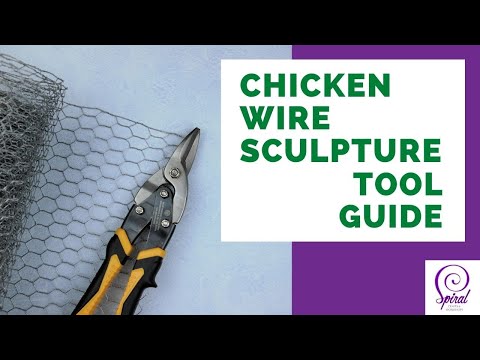The image serves as the title for a blog post or video and features a well-defined layout. Dominated by a background image on the left side, the image reveals a pair of metal pliers with yellow and black handles, resting on a white background with chicken wire. This scene visually suggests the topic revolves around sculpting tools. The right side of the image is filled with a solid purple color, providing a stark contrast to the left. Across the image, a white box with green text in all caps reads "CHICKEN WIRE SCULPTOR TOOL GUIDE," clearly indicating the purpose of the content. Additionally, the bottom right corner showcases another white box with the word "SPIRAL" in purple text, featuring an ornate "S" that curls into a spiral above the remaining letters. This detail adds a creative touch to the overall design. The use of long black horizontal bars at the top and bottom frames the image and adds an extra layer of emphasis to the central content.